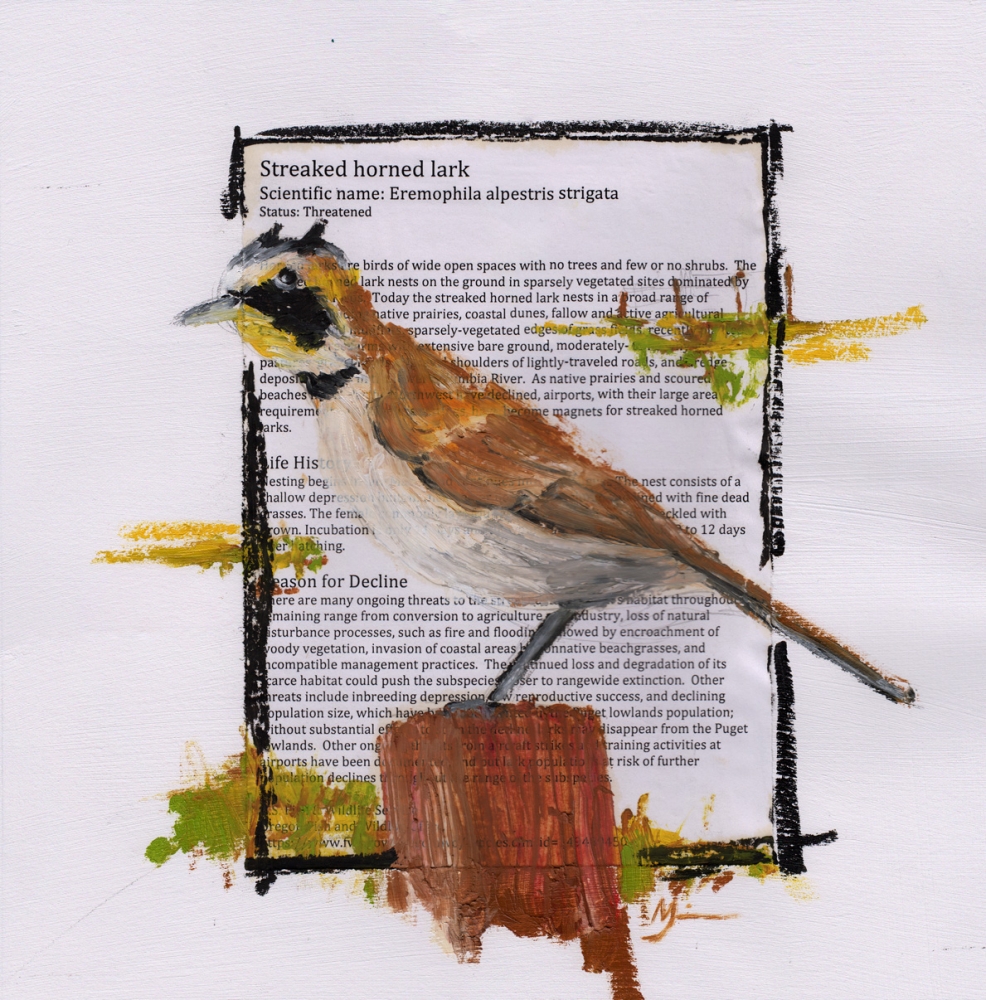The image captures a square watercolor painting of a streaked horned lark (scientific name: Eremophila alpestris strigata), identified as a threatened species. The background features an off-white piece of paper with black text, partially obstructed by the bird. The visible text at the top includes the bird's name and a brief description of its habitat, emphasizing wide open spaces with sparse vegetation and ground nests. The edges of the paper are outlined in black, possibly with charcoal or chalk, giving way to scribbles and smudges of yellow and green resembling tree branches and foliage.

The bird itself is perched on a brown tree trunk or stump, centrally positioned over the text. It displays a mix of colors: a yellow and black face, brown back, and a light tan to whitish underbelly with grey towards the legs. The bird has a greyish-yellow beak and grey legs. Surrounding the tree trunk are splashes of green and mustard, mimicking grass and possibly leaves, while the border of the image contains additional artistic strokes in similar colors, blending seamlessly into the composition.